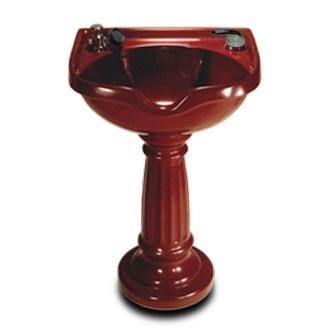The image depicts a detailed close-up of a modern, red pedestal sink set against a stark white background. The sink is characterized by its deep, burgundy red basin that features a prominent dip in the front for ergonomic hand placement. The base of the sink is round and leads up to a stemmed cylindrical column adorned with vertical grooves, reminiscent of a Roman column, and interspersed with small circular rings. These rings connect the column to both the round base at the bottom and the circular basin at the top. The sink appears to be made of porcelain with a glossy enamel finish. On either side of the back of the basin, there are mounted, metallic, silver handles that serve as water controls, but they do not extend upwards as traditional faucets do. This modern yet classical piece looks ideal for a stylish guest bathroom.